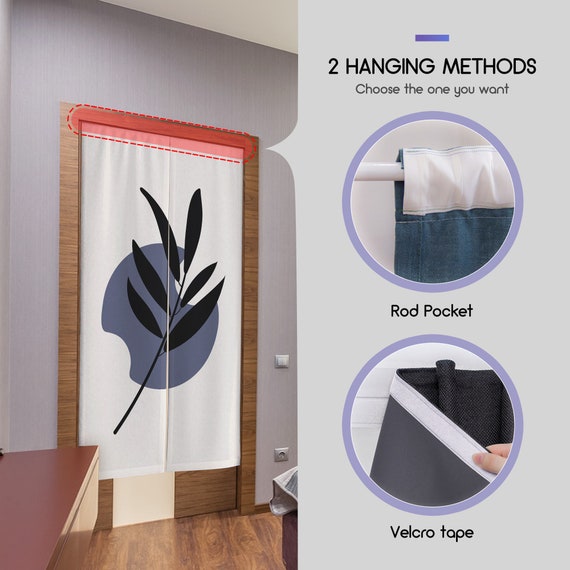This image displays detailed instructions for hanging a curtain featuring two distinct methods. On the left side, a white curtain adorned with a black plant design hangs in front of a brown-bordered door set against a violet-magenta wall. A blue circle intersects the curtain’s design where it splits. The top of the curtains is highlighted in red. On the right side, these instructions are set against a grey background, with a small purple rectangle at the top, followed by the two hanging methods you can choose from. The first method illustrates the curtain hung from a rod pocket, shown with a zoomed-in image of the curtain rod inserted into red pockets. The second method demonstrates attaching the curtain to the wall using Velcro, depicted with an image of Velcro tape.